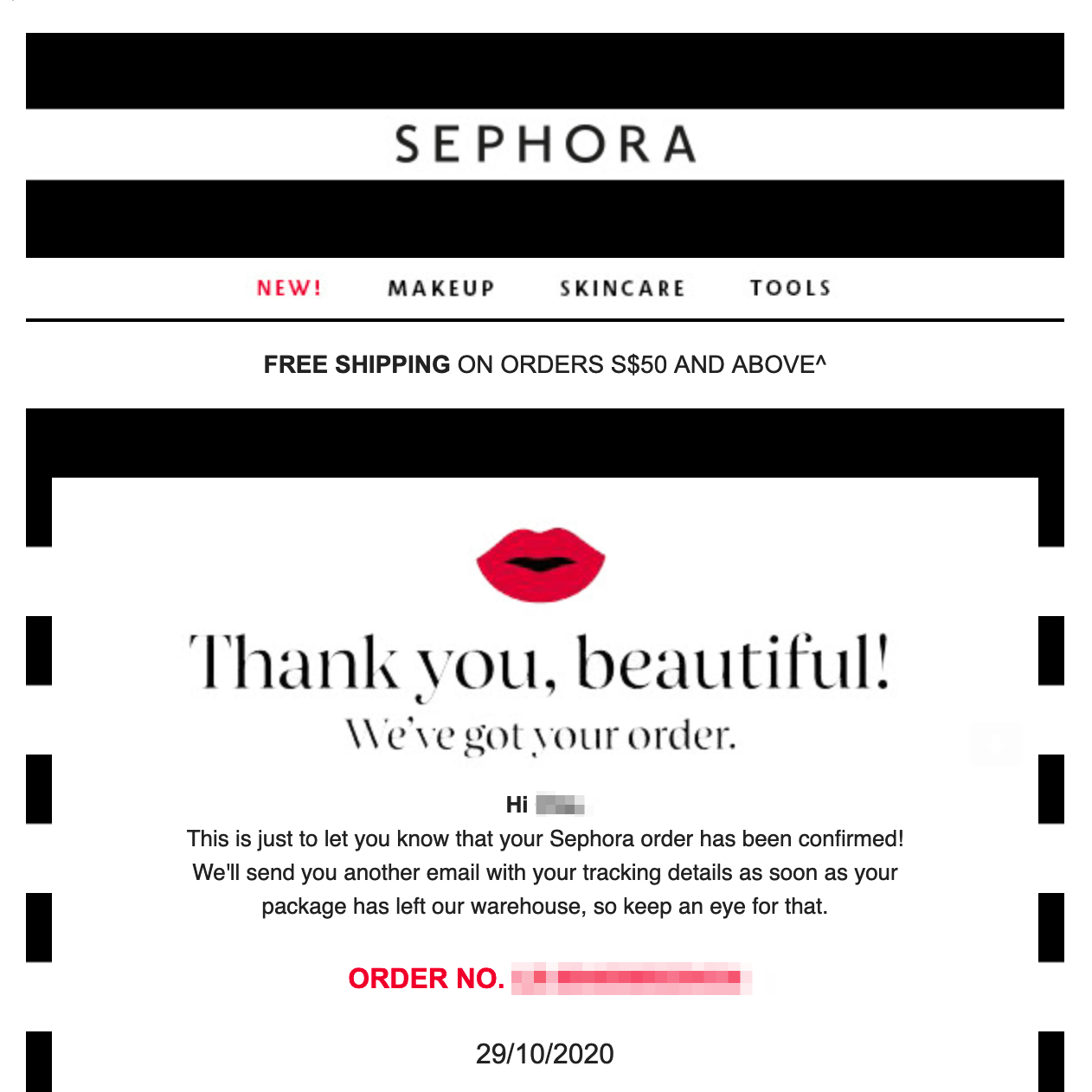This image is a detailed screenshot from the Sephora website, prominently featuring the brand's iconic black and white stripes. At the top, navigation tabs for "New," "Makeup," "Skincare," and "Tools" are clearly visible. A banner announces, "Free shipping on orders of $50 and above."

Below this section, the screenshot captures an email confirmation from Sephora. The email features a welcoming message that reads, "Thank you, beautiful!" with a graphic of red lips positioned above it. The text confirms the recipient's order with a friendly "Hi!" where the customer's name has been redacted for privacy. The message continues to confirm that the Sephora order has been successfully placed and promises another email with tracking details once the package departs the warehouse.

For added security, the order number is blanked out, and the date, October 29, 2020, indicates the email's original timestamp. Despite being from four years ago, this email format is likely still in use, serving as a reliable way for Sephora to keep customers informed.

The detailed email assures the recipient to keep an eye out for tracking information and provides a comforting reminder that their order is on its way. Regular Sephora shoppers appreciate these updates, as they provide peace of mind and enhance the overall shopping experience by keeping them well-informed about their order status.